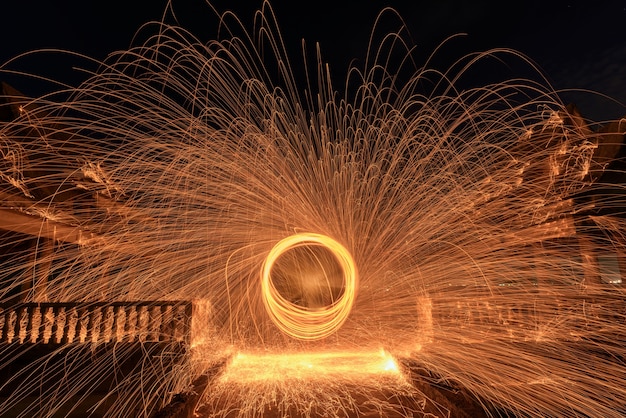The image depicts a mesmerizing light display reminiscent of fireworks or a spinning firecracker. At its center, a dazzling array of circular lights radiates outward, resembling a pinwheel with bright, sparkling trails captured in motion, creating intricate patterns that dominate the foreground. The dark night sky serves as a dramatic backdrop, enhancing the brilliance of the light show. Flanking the scene on either side are banisters, with decorative dragon-like figurines perched atop columns, adding an element of architectural flair. The bottom of the image is illuminated brightly, likely from the intense glow emanating from the center, and the setting appears to be an urban space, possibly a waterfront or downtown area, suggesting a celebratory event.